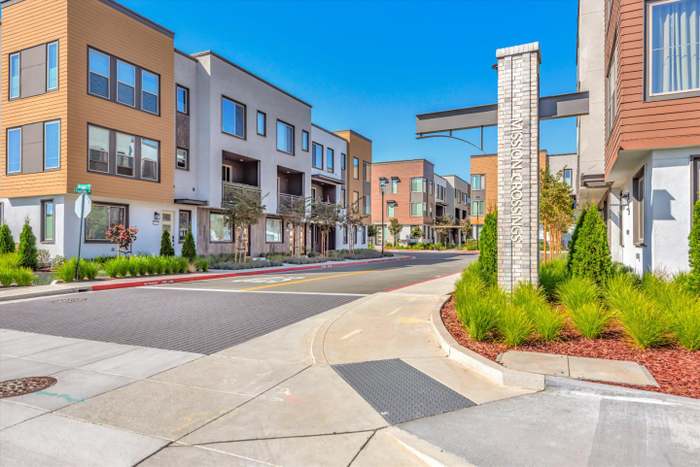This photograph captures a serene, modern suburban street scene taken from the perspective of a right-hand turn. The street has a clean, light gray pavement with yellow lines demarcating the center and a visible uncovered water hole. Clear blue skies provide a calm backdrop to the row of three-story, rectangular buildings lining either side of the street. These buildings are boxy and geometrical, with some sporting colors like orange, green, and dark brown, typically with off-white bases or stone accents. The structures appear interconnected, similar to row houses or apartment buildings, and are interspersed with flowerbeds showcasing green plants and mulch. Notably, there are four evenly spaced trees per block enhancing the greenery. On the right side, prominently in the foreground, stands a tall brick pillar on a red pebbled driveway with bushes, labeled "Mission Crossings" in white letters. In the background, the road splits off, further revealing more of this meticulously planned residential area.